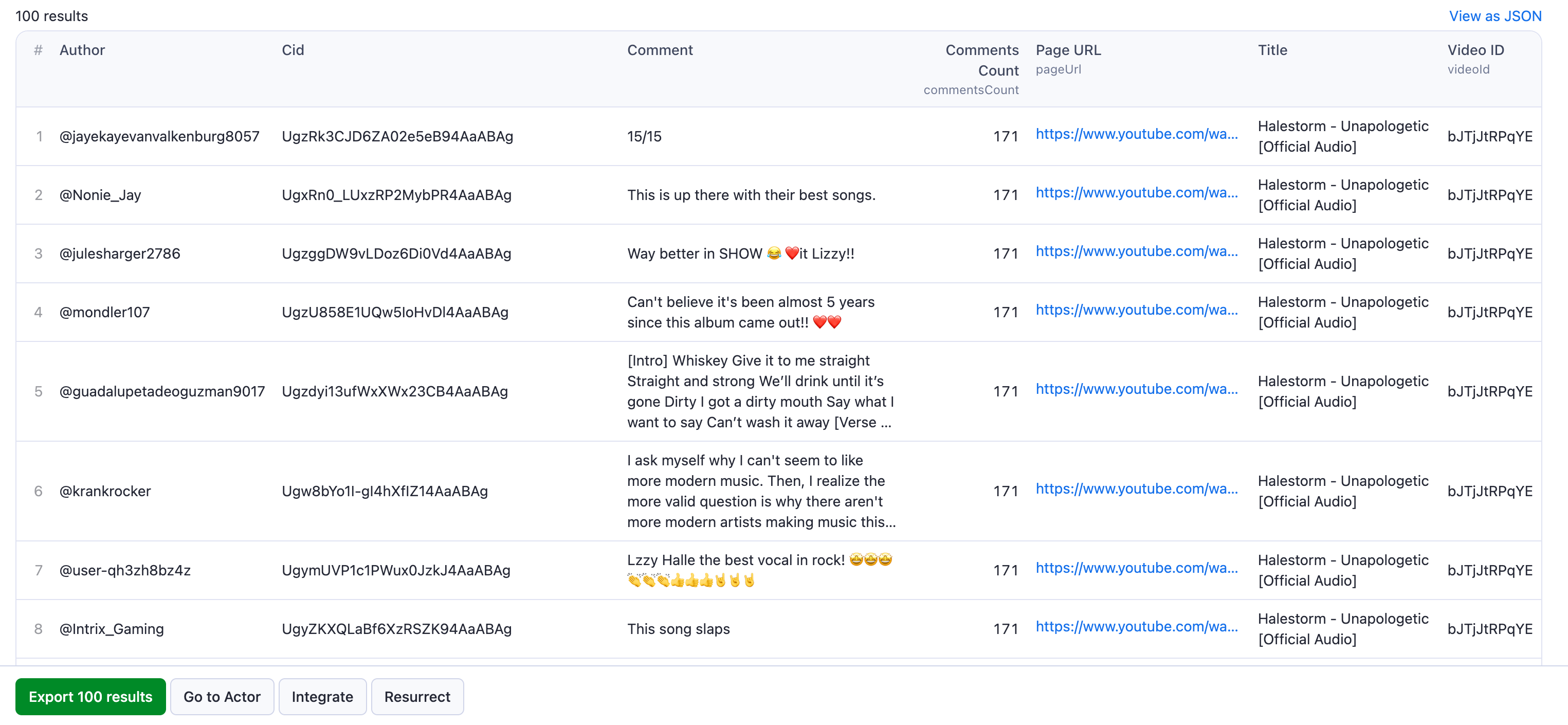A web page features an image showcasing a compilation of comments from eight different users about the song "Hail Storm Unapologetic." On the left side, usernames such as @Nonies_J and @JulieHarger are listed alongside their comments. Each comment reflects on the song's impact, with one user expressing disbelief that it's been almost five years since the album's release. The page resembles a YouTube comments section, with various users leaving feedback, including statements like "This song slaps" and emotive responses with heart emojis. Some comments mention that the song is among the best and recall attending a concert by the band, highlighting the enthusiastic and positive reception from all eight individuals.